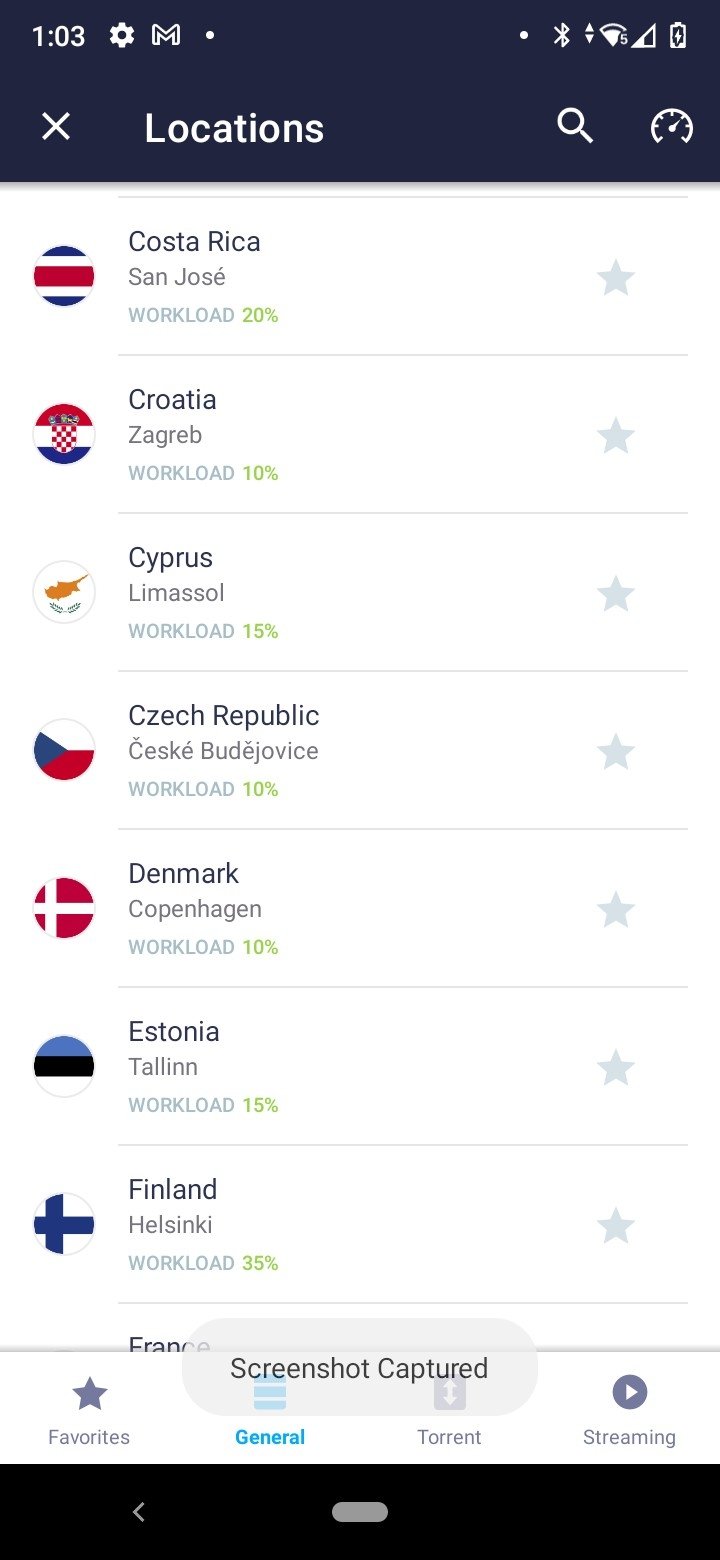This caption provides a detailed description of a screenshot taken from a smartphone app, likely used for torrent activities. 

---

The image showcases a smartphone screen with an unfamiliar app interface. At the very top of the screen is a clock displaying "1:03," alongside several icons: a gear (settings) icon, a Google Mail icon, a Bluetooth icon, a Wi-Fi signal indicator, a signal strength meter showing around 50%, and a battery meter indicating low battery.

Beneath this top bar, the screen displays the word "Locations" and features a search button with a magnifying glass icon. To the right of the search button is an icon resembling a speedometer, possibly related to download speed.

The bottom bar of the app provides navigation options labeled "Your Favorites," "General," "Torrent," and "Streaming," indicating that this is a torrenting application.

The main section of the screen lists various countries and cities along with their workload percentages, and each entry is accompanied by a gray star on the far right, none of which are marked. The top entry shows Costa Rica, San Jose with a workload of 20%. Following entries include Croatia, Zagreb (10%), Cyprus, Limassol (15%), Czech Republic, represented by a partially illegible city name (possibly "České Budějovice"), Denmark, Copenhagen (10%), Estonia, Tallinn (15%), and Finland, Helsinki (35%).

This detailed breakdown clarifies that the app is listing torrent server locations and their current workloads.